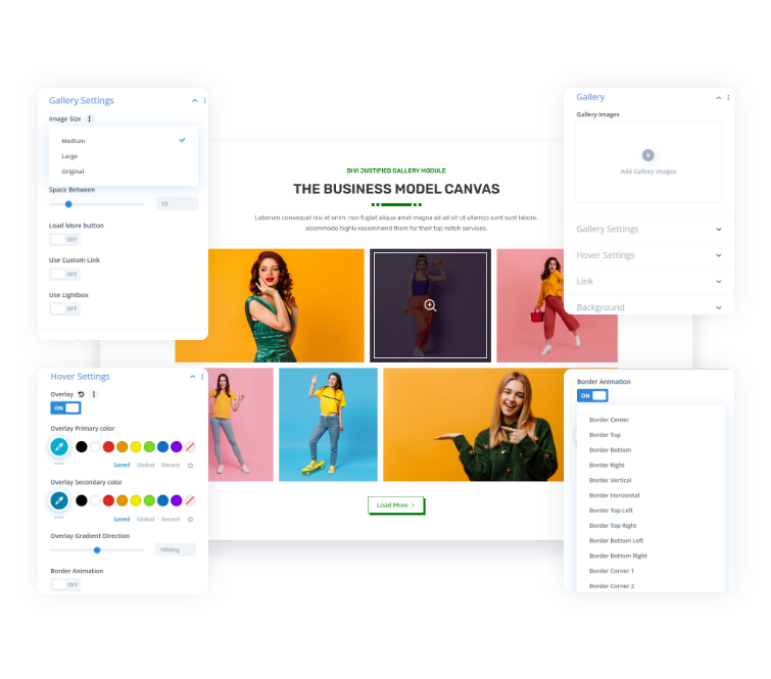This image is a detailed collage featuring a central primary image flanked by four smaller pop-up images in each corner. 

The central image has a white background adorned with green text at the top that reads "Divi Justified Gallery Module, the Business Model Canvas." Surrounding this text are various images of young women posed against vibrant, colorful backdrops including shades of yellow, purple, pink, blue, and again yellow. Specific details in this central image include a woman with red hair, green dress, red makeup, and red lipstick. Two of the women sport blue jeans paired with yellow shirts, while another is dressed in a green sweater with blonde hair styled to the side. A "Load More" button is centered at the bottom of this primary image.

Each corner features a pop-up image with distinct settings menus and options:
- In the top left corner, the pop-up titled "Gallery Settings" includes configuration options such as Image Size (with "Medium" selected), Space Between (set to 10), "Load More Button" and "Use Custom Link" both toggled off, and "Use Lightbox" turned off. Below are "Hover Settings" with "Overlay On," featuring color options and an overlay gradient direction controlled by a slider.
- The top right corner pop-up, labeled "Gallery Images," allows users to add images to the gallery. It also refers to "Gallery Settings," "Hover Settings," "Link," and "Background" configurations.
- The bottom right corner contains a pop-up for "Border Animation," which is toggled on. It presents various options for border customization including center, top, bottom, right, vertical, horizontal, top left, top right, bottom left, bottom right, corner one, and corner two.

This immersive layout encapsulates a comprehensively detailed visual offering multiple customization options for creating dynamic and visually enticing galleries.